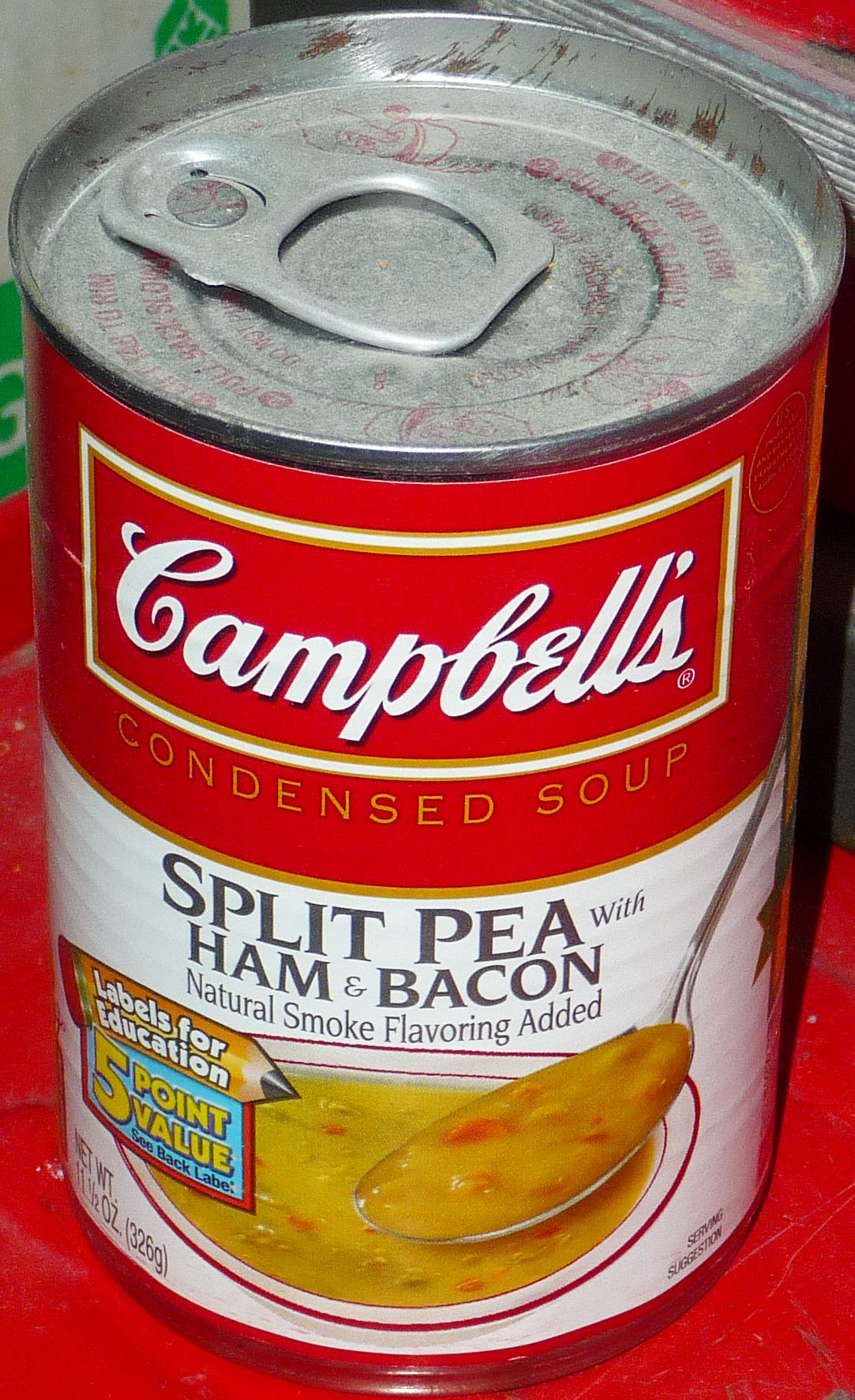This indoor color photograph features a single can of Campbell's Split Pea with Ham and Bacon Condensed Soup, resting on a red countertop. The perspective is a three-quarter view looking down at the can, which appears somewhat dusty, suggesting it has been in storage for a while. The can is unopened, with its metallic tab pointing toward the upper left corner.

The label is the classic Campbell's design: the upper third is red with white cursive "Campbell's" lettering, and just below that, in gold or orange capital letters, it says "Condensed Soup." The lower two-thirds of the label are white, displaying the soup type in bold black capital letters: "Split Pea with Ham & Bacon," followed by "Natural Smoke Flavoring Added." There is a realistic image of a ceramic bowl filled with the soup, with a silver spoon lifting a portion from the bowl, positioned to the right side of the image.

On the left side of the label, there's an additional overlay showing a pencil lying on its side. This part of the label is marked "Labels for Education" in white, with a yellow "5 Point Value CBAC Label" sign beneath it. The can is true to its iconic, traditional look, emphasizing both its brand and the detailed depiction of the soup within.